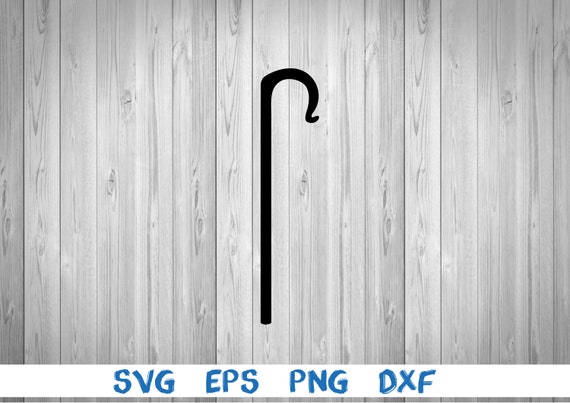The image features a black hook-like object resembling either a cane or a rod, which stands vertically and then curves to the right at the top. This object is positioned against a background of vertical wooden planks, giving the appearance of a wooden wall or fence characterized by its grain marks and line details. The scene is set in grayscale, making the black object stand out prominently. At the bottom of the image, a white stripe runs horizontally, serving as a backdrop for blue text that reads "SVG EPS PNG DXF," presented in a format similar to a television chyron. These letters are graphic file formats, although no specific context is given for their appearance in the image.